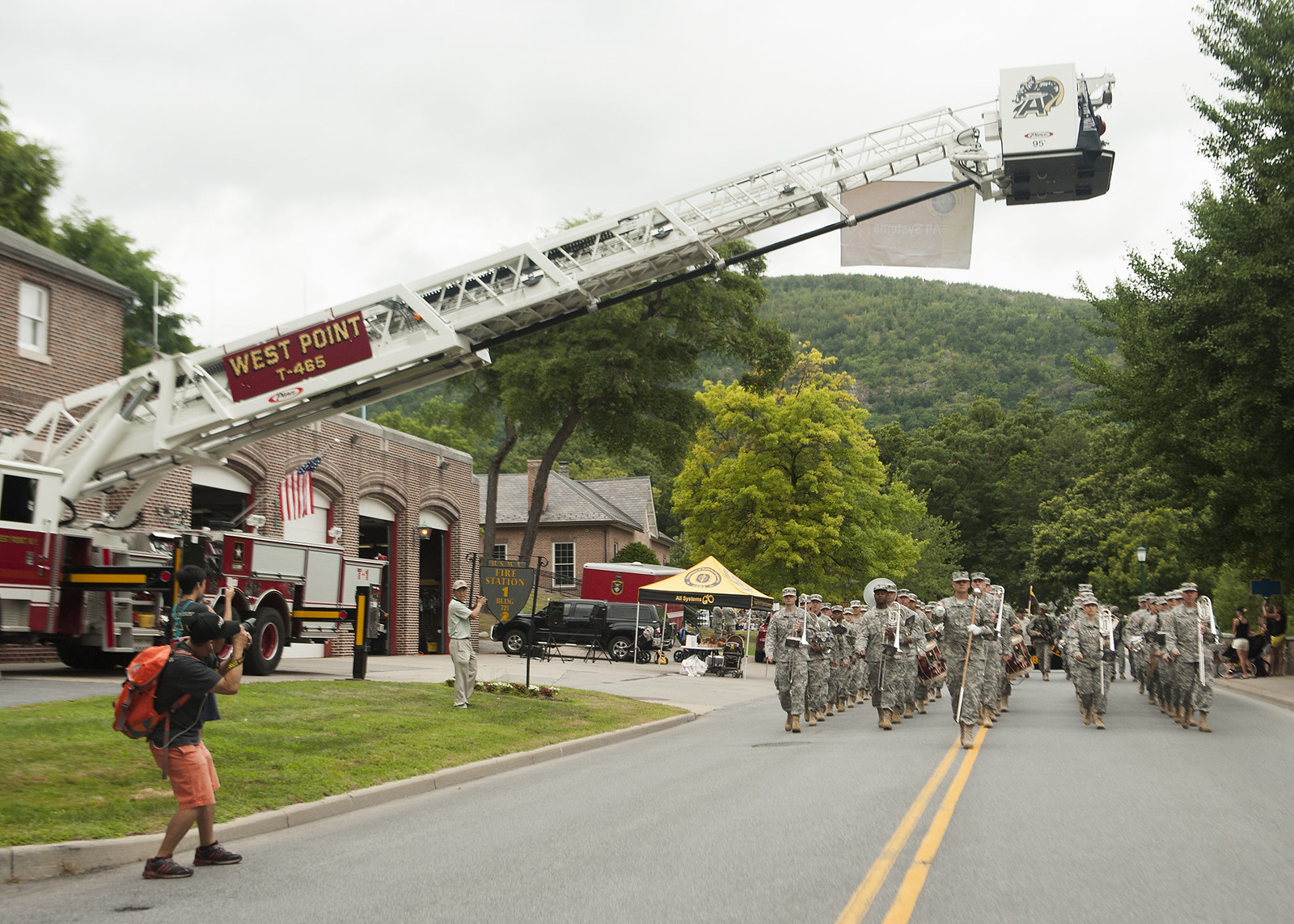The photograph captures an outdoor scene at West Point featuring a parade of army soldiers marching in formation down a road. The soldiers are organized into straight, orderly lines with some holding musical instruments such as tubas, suggesting a ceremonial parade. The parade is framed by a picturesque backdrop of a green mountain and lush trees, indicating a natural, scenic environment.

On the left side of the image, a brick fire station is prominently visible with its doors open and an American flag displayed. A large fire truck is parked in front of the station, its ladder extended out over the road, and the words "West Point T465" are visible on the boom. In front of the firehouse, there is a booth set up next to a black truck, and a sign reading "Fire Station 1" which a man appears to be installing.

Spectators are gathered on the right side of the road, including a man in orange shorts and a black shirt with an orange backpack, who is taking pictures of the event. Near the tents set up by the fire station, other onlookers can be seen, some holding instruments or sticks. The scene is lit by daylight, though the sky appears cloudy and foggy, adding a soft, diffused light to the setting.